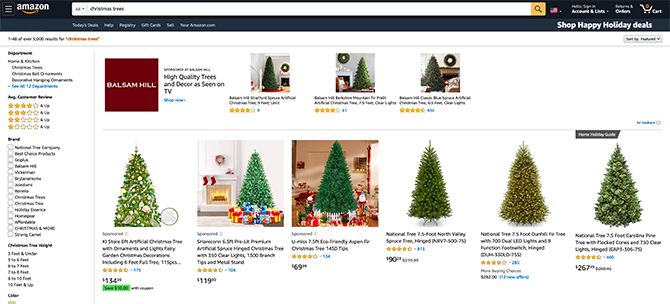This is a detailed screenshot from Amazon.com, featuring search results for "Christmas trees." In the upper left corner, the Amazon logo is prominently displayed in white with the characteristic yellow arrow beneath it. The search bar indicates that "Christmas trees" were entered, yielding various results along with an advertisement for Balsam Hill, which boasts high-quality trees and decor as seen on TV.

At the top of the results, there is a highlighted section showcasing three Christmas trees, all from Balsam Hill. These trees appear plush and well-constructed, though they are artificial. Each tree has a traditional triangular shape and a rich dark green hue. The ratings for these Balsam Hill trees are notable, with two receiving four stars and one earning four and a half stars.

Below this highlighted section, six more Christmas trees are displayed. The ratings for these trees are consistently high, with one tree receiving four and a half stars while the others range between four stars and slightly above four stars. As with the Balsam Hill products, these trees also feature a classic triangular shape and dark green color, making them visually appealing choices for the festive season. Overall, the selection offers a variety of highly-rated, artificial Christmas trees suitable for holiday decor.